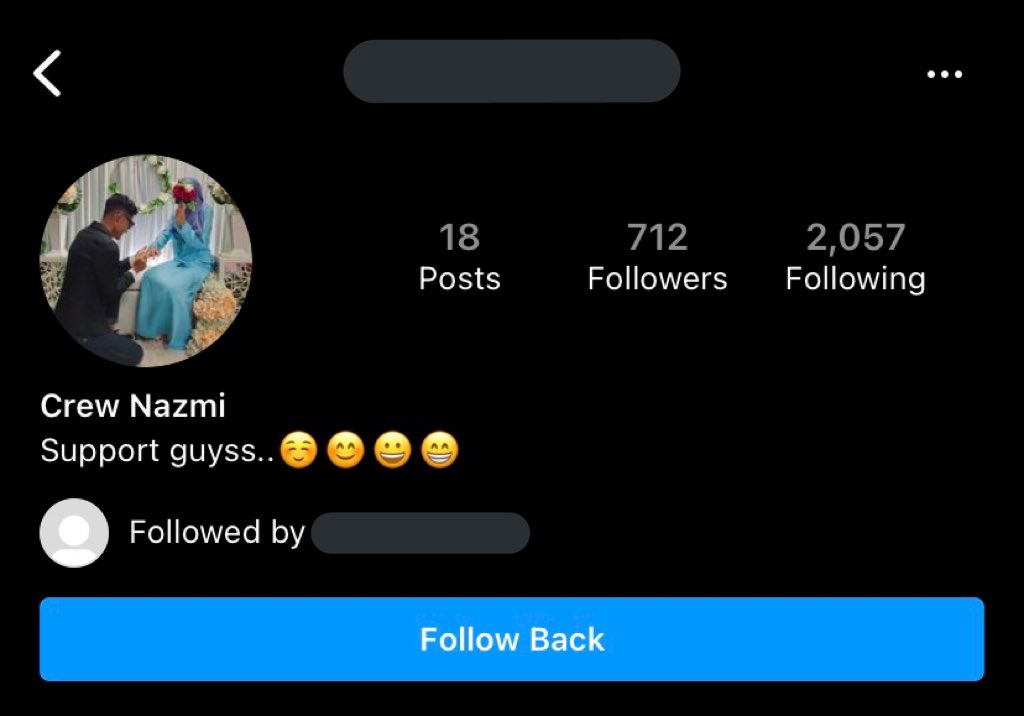This image captures a Twitter profile belonging to an individual named Kru Nazmi. The profile picture features a romantic scene where a man is bending down, seemingly placing a ring on the finger of a woman dressed in a long dress and a headscarf. The backdrop appears to be a white room adorned with flowers, and the woman is visibly emotional, covering her face with one hand while extending the other. The account details reveal that Kru Nazmi has made 18 posts, has 712 followers, and is following 2,057 people. Below the profile information, there is an indication that the account is followed by someone, although the name is obscured. Additionally, a large blue button labeled "Followed Back" is prominently displayed.